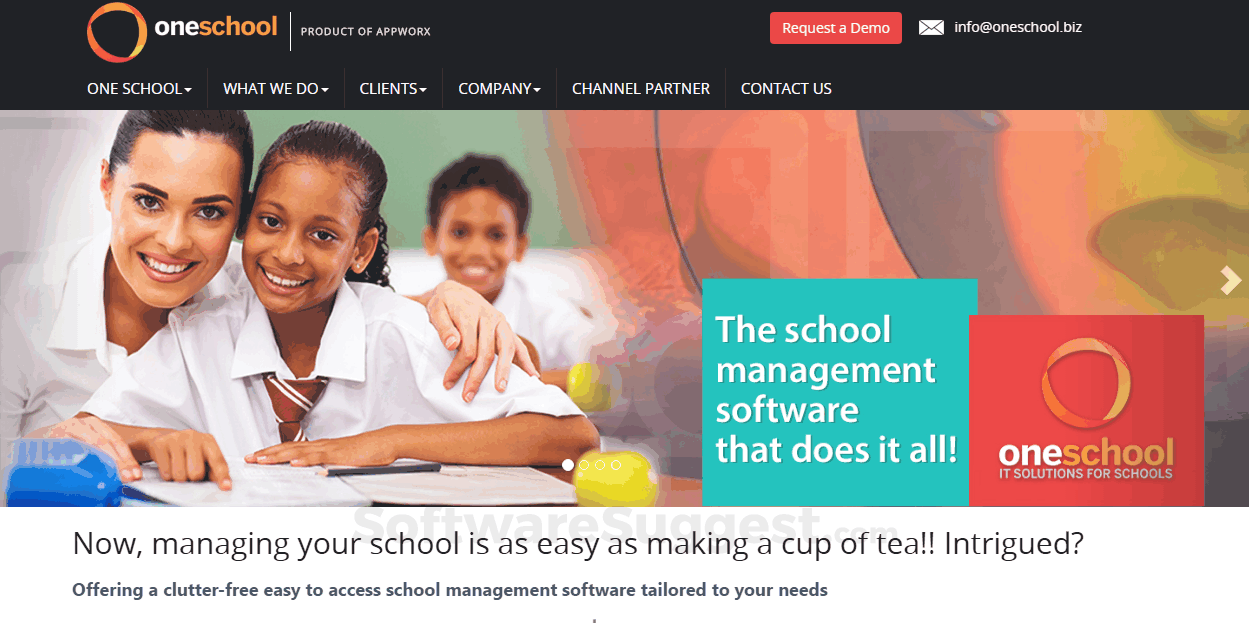**Panoramic Image Caption:**

At the top of the panoramic image, there is a long black navigation bar containing several elements. On the upper left, there is an orange and yellow circle with a black center. To its right is white text that reads "C1," followed by orange text that completes the phrase as "School." 

Right next to this is a thin white vertical line, followed by white capitalized text that states, "This is a product of AppWorx." Towards the far right of the black bar, there is a red box with white text that reads, "Request a Demo," and an envelope icon next to it. Further right is an email address in white text: "info@oneschool.biz."

Beneath this bar is a clickable white menu in all capital letters, from left to right: 
- "One School" with a clickable icon beside it
- "What We Do" with a clickable downward-facing triangle
- "Clients" with another clickable downward-facing triangle
- "Company" with a clickable downward-facing triangle
- "Channel Partner" without a menu, just clickable text
- "Contact Us," also without a menu.

In the main body of the image, we see what appears to be a classroom setting featuring two women—one presumed to be a teacher, who is African American, and a student possibly of African or Indian descent. Both women have long black hair and are dressed in white shirts. The student is seated with papers and a gray pen in front of her, with the teacher standing beside her, placing her arm around the student's shoulder in a nurturing gesture. Above the teacher's arm, another student with short black hair and a white shirt is visible in the background, but this figure is much blurrier.

The background of the scene, particularly towards the right, is a mix of pink, purple, and yellow hues. On the lower right, there is a teal-colored square with white text that reads, "The school management software that does it all." Overlapping this square is a red rectangle containing the orange and yellow logo from the upper left corner. In the center of the red rectangle, the words "One School" are written in white and orange text. Below this, gray capital letters spell out, "IT solutions for schools."

Towards the far right, a large white sideways-facing "V" shape is present, and beneath it, there is a faint watermark in gray lettering that reads, "SoftwareSuggest.com." Positioned above this watermark is black text stating, "Now managing your school is as easy as making a cup of tea. Intrigued?" Below this, in a slightly different shade of gray text, the statement continues, "Offering a clutter-free, easy access to school management software tailored to your needs."